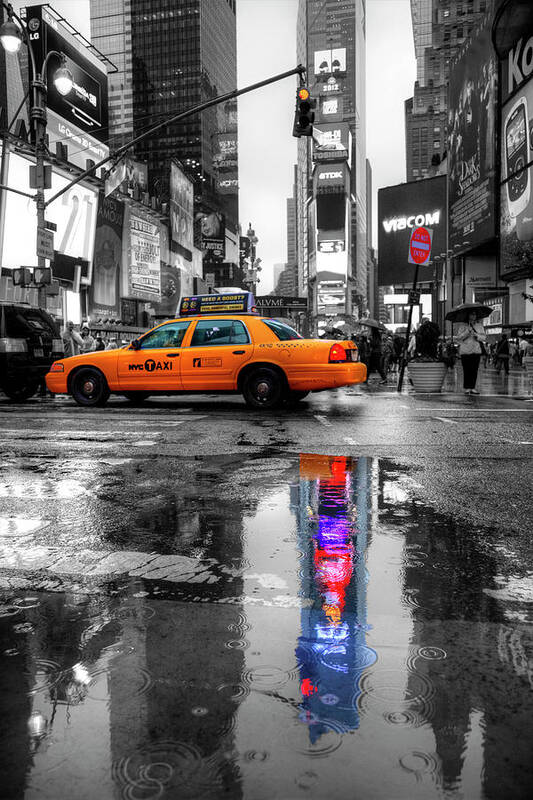In this detailed and captivating photograph of New York City, we see a prominent yellow taxi cab, a striking burst of color amidst a predominantly black and white scene. The taxi occupies a central position, either parked or in transit, adding a vibrant contrast to the grayscale surroundings. Above the taxi, a yellow traffic light hangs, contributing to the color dynamics along with a visible "Do Not Enter" sign.

The scene is set on a rainy day, evidenced by the large puddles on the street. One puddle, in particular, captures the reflection of a high-rise building with its LCD screens in full color, even though the actual building in the frame is in black and white. Similarly, the rest of the high-rise buildings and the people on the street are rendered in grayscale, emphasizing the artistic color contrast of the photograph.

Overall, this artsy image captures the bustling essence of New York City, potentially Times Square, with its unique play on color and monochrome elements, creating a visually striking and atmospheric portrayal.